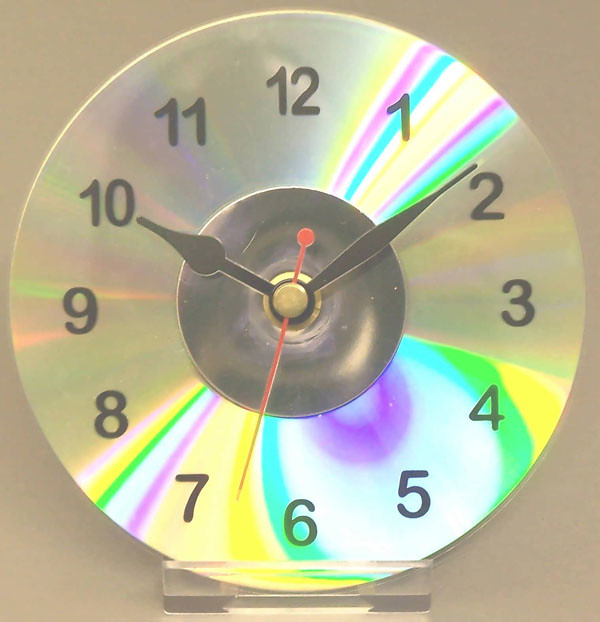This photograph features a slightly taller-than-wide square image of a unique, retro-inspired clock crafted from an old-fashioned compact disc (CD). The CD serves as the clock face, adorned with the numbers 1 through 12 to mark the hours. The clock's hour and minute hands are black, while the second hand stands out in red, sweeping smoothly across the surface. 

The CD displays a captivating rainbow iridescence, a characteristic trait of CDs, with the most vivid colors appearing near the 1 o’clock position and between the 7 and 8 o'clock marks. Additional shimmering hues can be observed between the 3 and 8 o’clock positions, contributing to the overall kaleidoscopic effect on the CD.

This colorful timepiece is mounted on a lucite base, giving it a modern touch, while the entire scene is set against a warm tan or beige background, allowing the vibrant colors and unique design of the CD clock to stand out prominently. The whimsical nature of this clock adds a playful and nostalgic charm to the photograph.